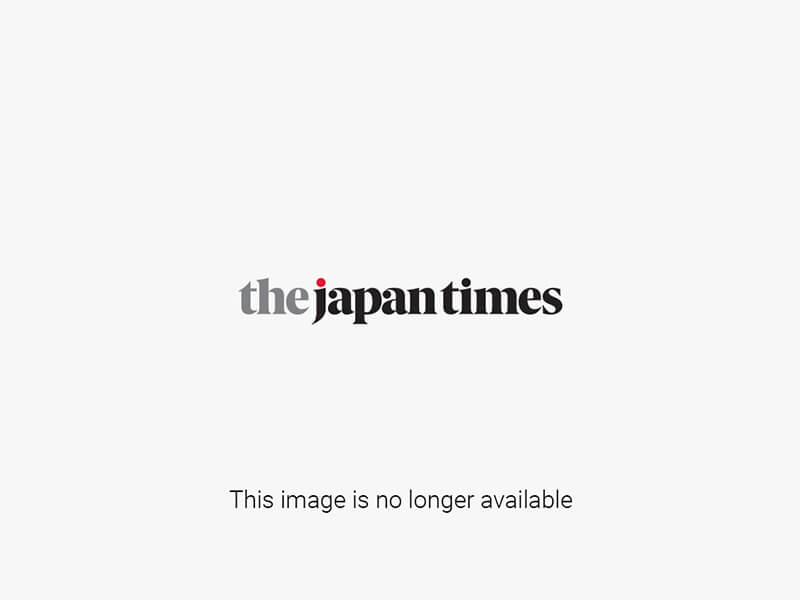The aerial photograph captures a densely built-up metropolitan area, with numerous buildings sprawling across the background and diagonally along the right-hand side. At the center of this urban landscape is a striking, large green area dominated by vibrant, leafy trees. This green zone is uniquely shaped like a keyhole— an extraordinary design feature that includes a large man-made cutout resembling a lock. Encircling this keyhole-shaped grove is a body of water, appearing mint-green in color in the photograph. Surrounding the water, there's an additional ring of lush trees, enhancing the central keyhole shape. The entire scene is bathed in daylight, highlighting the vivid greenery and the intricate, lock-and-key pattern that is only visible from this aerial viewpoint.